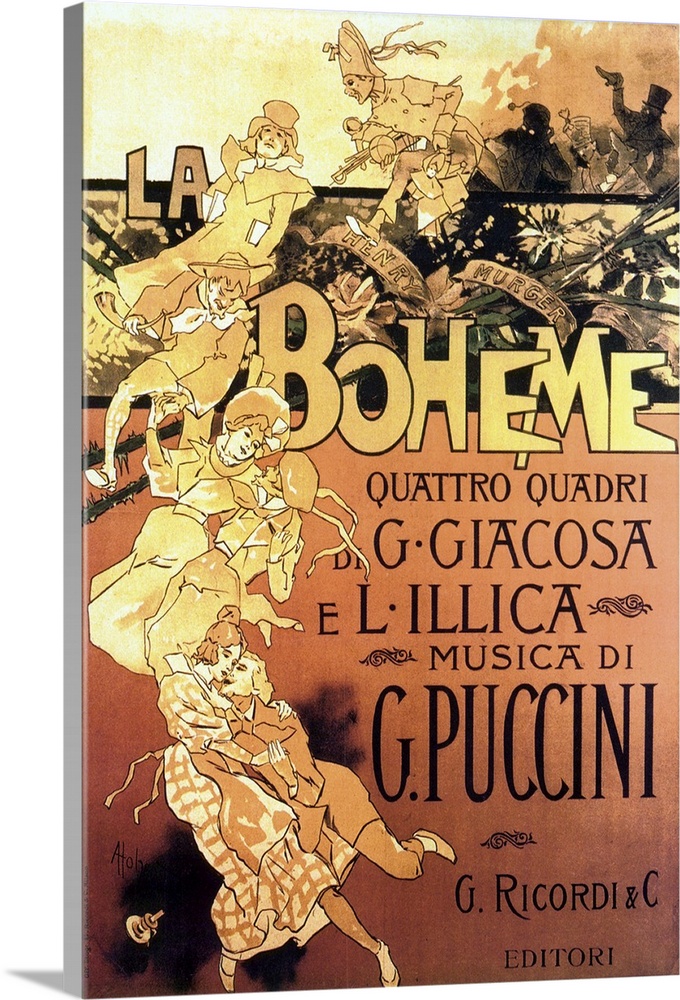This image appears to be advertising material for La Boheme, either a book cover or a poster. The top third of the image features an intricate outline drawing of various people, showcasing an 18th-century European aesthetic. Among these figures, one notable character is a person wearing a French revolutionary hat, carrying an assortment of objects including a doll, a ball, and possibly a sword. Surrounding this character are men in suits and top hats, women in dresses, and other individuals donning knickers. The drawing style is reminiscent of a pencil illustration.

Below the characters, the middle section of the image displays a close-up of a bouquet of flowers tied with a ribbon that reads "Henry Mercer" or "Mercer." 

Dominating the lower portion of the image, the title "La Boheme" is prominently written in a yellow font with a black outline. Below this title, in Italian, it states "Quattro Quadri by G. Giacosa e l'illica musica di G. Puccini," indicating the opera's authors and composer. The bottom section of the image has an orangey-pink color and includes the text "G. Ricordi and C. Editori." The overall design combines elements of color and black-and-white illustrations, with noticeable orange hues, creating an old-timey appearance that evokes the 1800s or earlier.